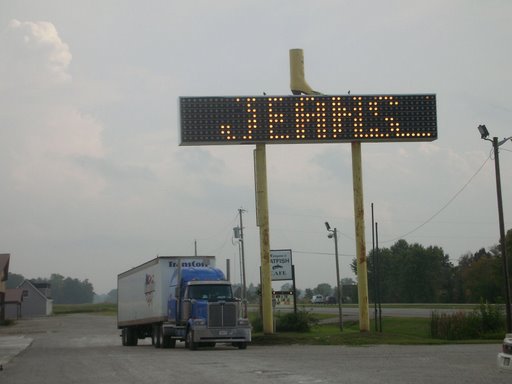In this outdoor photograph, a blue semi-truck with a sleeper cab and a white box trailer is the focal point, situated in a rural or semi-rural parking lot. The semi-truck is stationed next to a large, black reader board sign with brightly lit orange text that spells out "JEANS." Two tall, yellow poles support the sign, further emphasized by a yellow pipe above it. The scene includes some additional details such as power lines with lights, a glimpse of a small highway to the left, and a tip of a car's trunk and tail light visible in the bottom right corner. In the background, there are scattered buildings, possibly a truck stop or similar establishment, and a landscape featuring trees and a cloudy sky. The photograph captures both the tranquility of the rural setting and the presence of human-made structures, with the "JEANS" sign being a key point of interest.